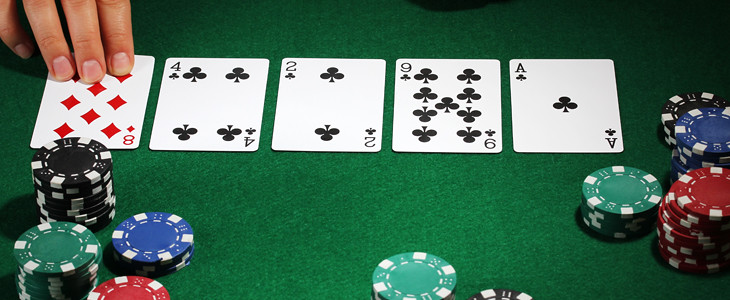The photograph captures a vibrant scene set on a green felt surface resembling a poker or blackjack table. In the left corner of the image, there are neatly stacked poker chips in green, blue, red, and black, with the black stack towering above the rest. Dominating the center of the composition, five playing cards are laid out sequentially from left to right: a red eight of diamonds, a black four of clubs, a black two of clubs, a black nine of clubs, and a black ace of clubs. Near the bottom center of the frame, there is a smaller stack of green and black chips visible. On the right side of the image, another stack of chips is observed, with the red and blue chips forming the tallest piles, each approximately nine to ten chips high. An aspect of human interaction is also present, as a hand—presumably that of a player—lifts the eight of diamonds card, indicating an ongoing game. This scene is likely taking place at a casino dealer's table, where the hand actively participates in the game atmosphere.